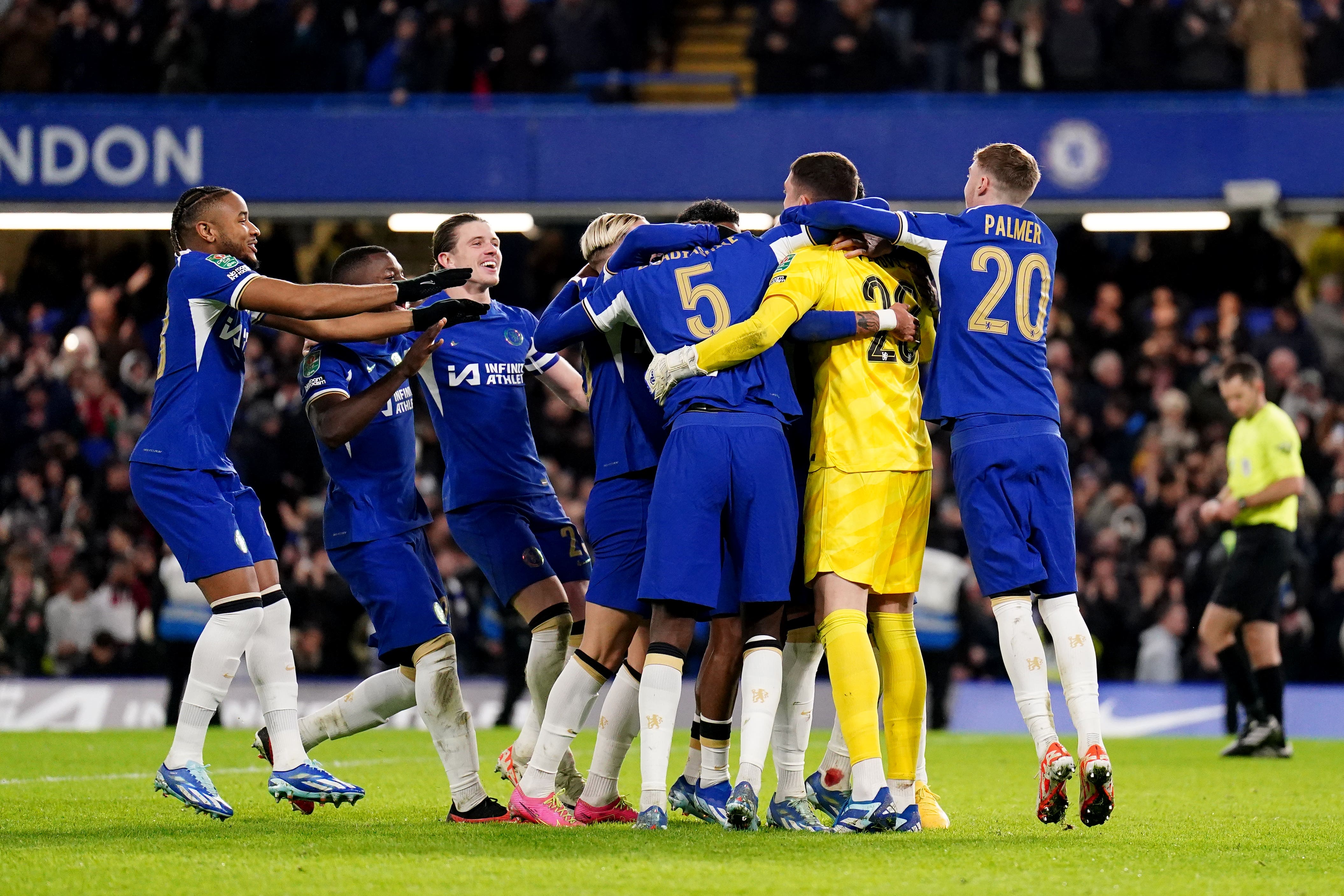This photograph captures the jubilant moment of a youth soccer team, likely celebrating a victory. The team predominantly wears royal blue uniforms, with visible numbers 5 and 20. The player wearing the number 20 jersey, named Palmer, is seen leaping into the group for a hug from behind, displaying vibrant joy. The front of their shirts showcases the logo and text "Infinite Athlete." Amidst them is a solitary player in a yellow uniform, possibly the goalie or a player from the opposing team, creating a striking contrast.

Standing out in the background is part of a stadium full of enthusiastic spectators, with the letters "L-D-O-N" prominently displayed on the balcony level, suggesting the location might be London. The image also shows a coach or referee in black shorts, a yellow top, and black shin guard stockings on the right side, adding to the bustling post-game environment. The diversity among the team members is apparent, with players of different races and hair colors wearing varied soccer cleats and shin guards, some appearing delightfully dirtied from the match. The scene is energizing, with blurred but crowded stands reflecting the excitement shared by fans and players alike.